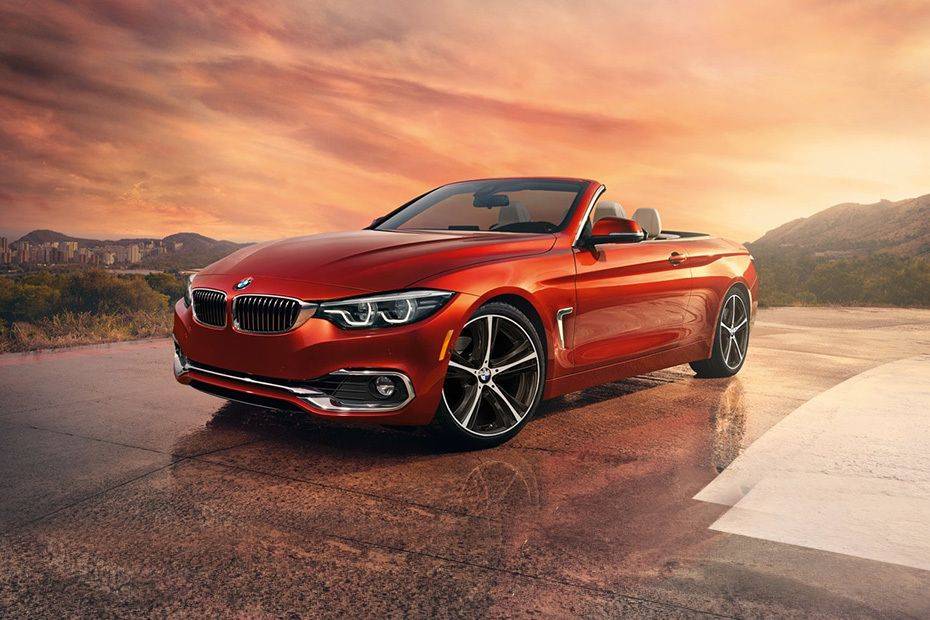The image features a modern, two-door BMW convertible with a sleek reddish-orange paint job, parked on a semi-reflective, wet concrete surface that appears to be stone or marble-like with dark splotching. The car, notable for its distinctive BMW center emblem and five-spoke wheels, boasts a white interior with the seats just visible. The surroundings include a semi-arid environment with grassy areas and shrubbery. To the right side of the image, a large mountain is visible with trees in front of it, while the left side shows more greenery and additional distant mountains. Below these mountains, in the far background, there's a visible cityscape. The sky above is filled with gray clouds, suggesting that the photo was taken during or after sunset. Overall, it's a picturesque setting for showcasing a very nice, modern BMW sports car.